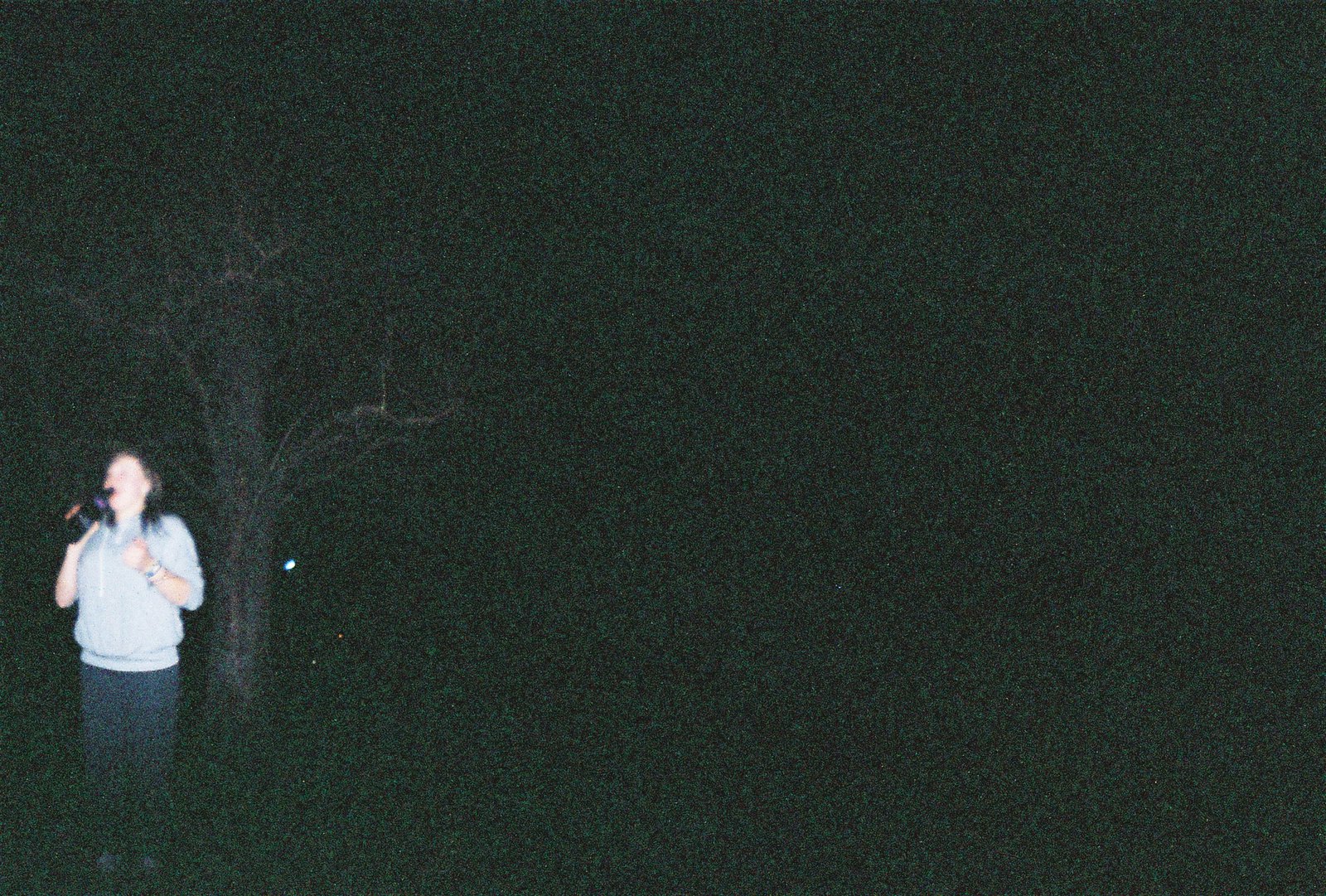In the foreground of this night shot, the stark flash of the camera illuminates a woman positioned in the bottom left corner. She stands facing forward, with medium-length brown hair cascading over her blue blouse and blue pants. In her left hand, she clutches a large bottle, resembling either wine or liquor, as she takes a drink. Her right hand is brought up towards her chest. Behind her looms an eerie, leafless tree with thin, twisted branches, adding a spooky element to the scene. The background is engulfed in complete darkness, save for a tiny, solitary white dot far in the distance to the right of the tree, further emphasizing the night setting.